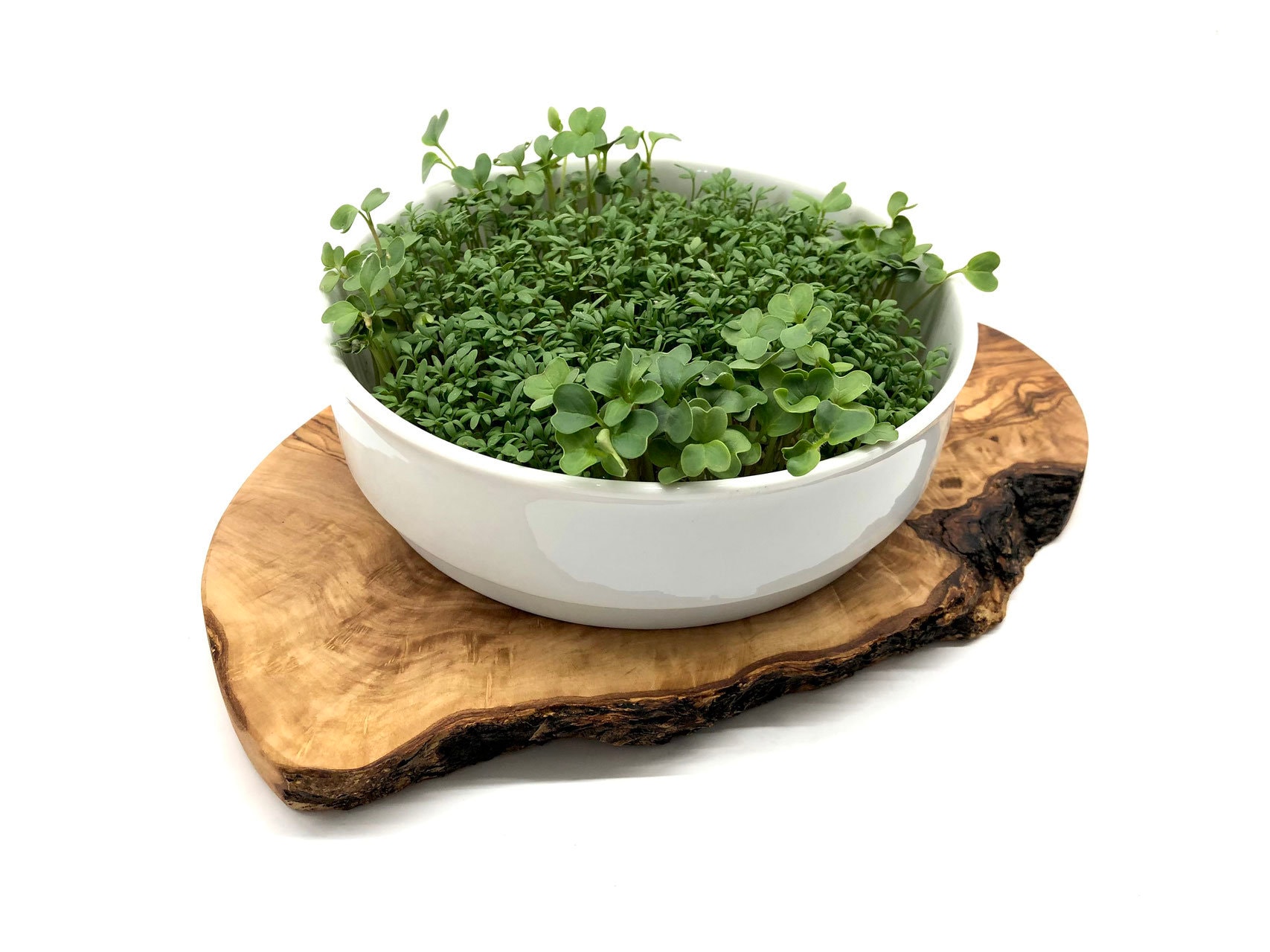A white ceramic bowl, boasting a slightly reflective sheen, sits centrally atop a rustic, unfinished wooden slice, which appears to have been freshly cut from a tree without any shaping or finishing. Inside the bowl, there's a dense collection of green vegetation, primarily resembling three or four leaf clovers. The tiny plants give the impression of a miniature, uncontrolled jungle spilling over the bowl's edges. The foliage varies in size and some leaves cascade over the rim of the bowl, emphasizing the vibrant and lush nature of the plants. The overall scene is set against a plain white background, with no other objects or people present, allowing full focus on the earthy, natural elements captured in the image.